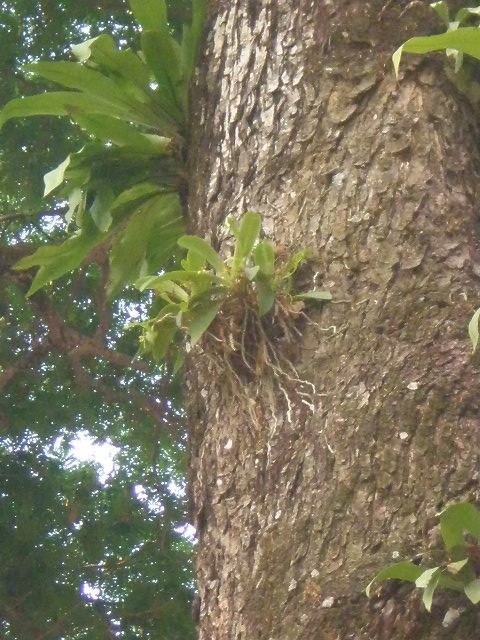The image captures an up-close view of a tree trunk that occupies most of the right-hand side of the frame. The bark, textured with grooves and lines, appears mottled with white speckles and features a light patch at the top, possibly illuminated by sunlight. Emerging from the trunk are several green plants, contributing to a lush, verdant look particularly concentrated toward the upper left of the tree. On the left side of the photograph, the view shifts upward, revealing the canopy of surrounding trees. Here, green leaves merge into a bright, blue sky, with sunlight filtering through the gaps. No people or text are visible in this vivid, natural outdoor scene.